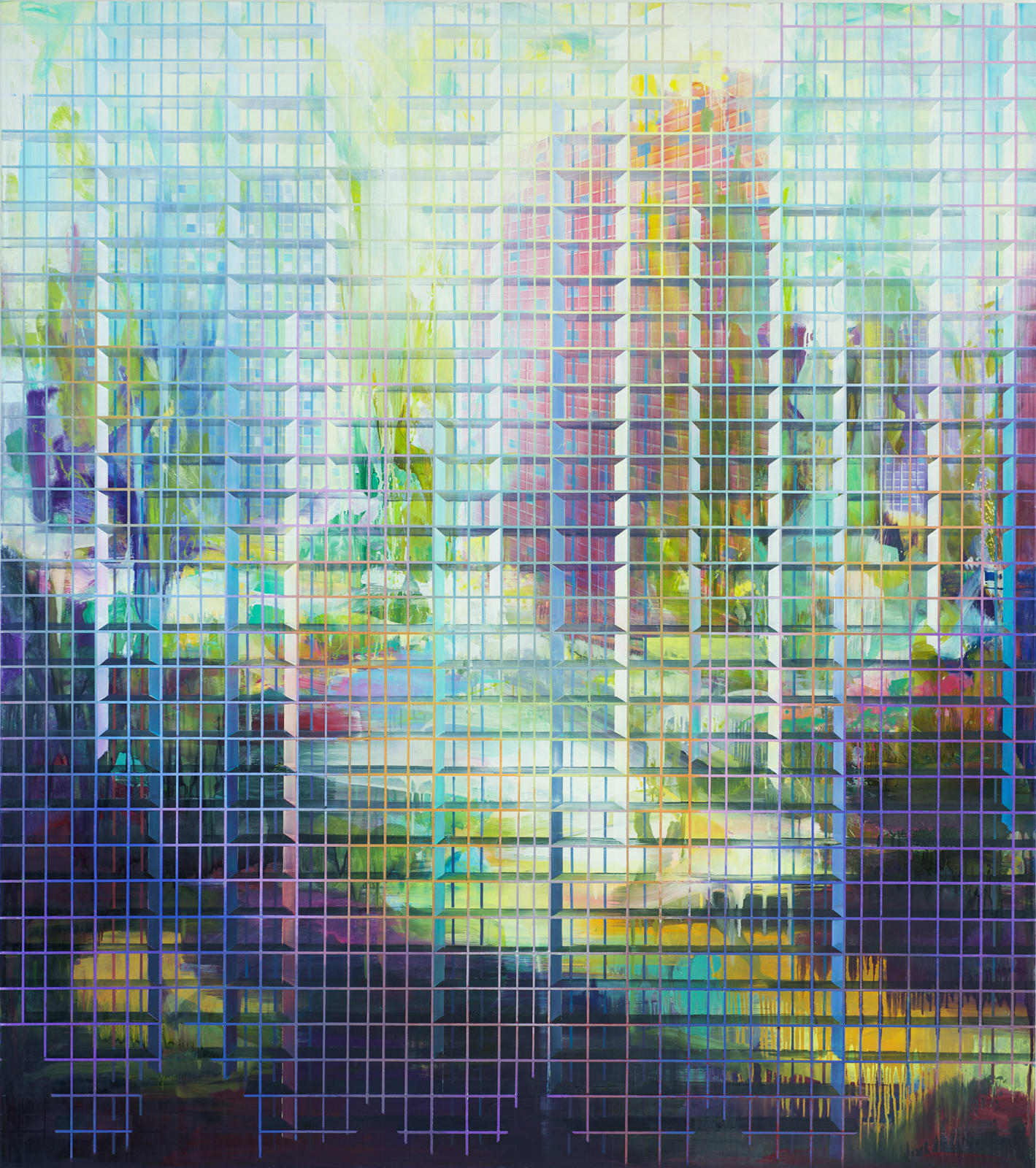The image appears to be an artist's abstract rendering, possibly digital art, resembling the side of a building with a reflective glass facade. The artwork is predominantly square-shaped, slightly taller than it is wide, and features a grid of small, pixelated squares created by an intersection of horizontal and vertical lines. This grid mimics the structure of windows on an office building. The color palette transitions from dark, earthy tones—such as black, browns, and purples—at the bottom, blending into reds and yellows. These darker hues suggest a shadowy or lower-light area, possibly reflecting a tree-planted street scene. Moving upward, the colors graduate into lighter shades, including greens and sky-blue tones, indicating a transition towards a lighter, more illuminated area influenced by a light source at the top. The overall effect is a complex mosaic of intersecting lines and varied colors, giving an impression of a pixelated, stylized reflection on a building.